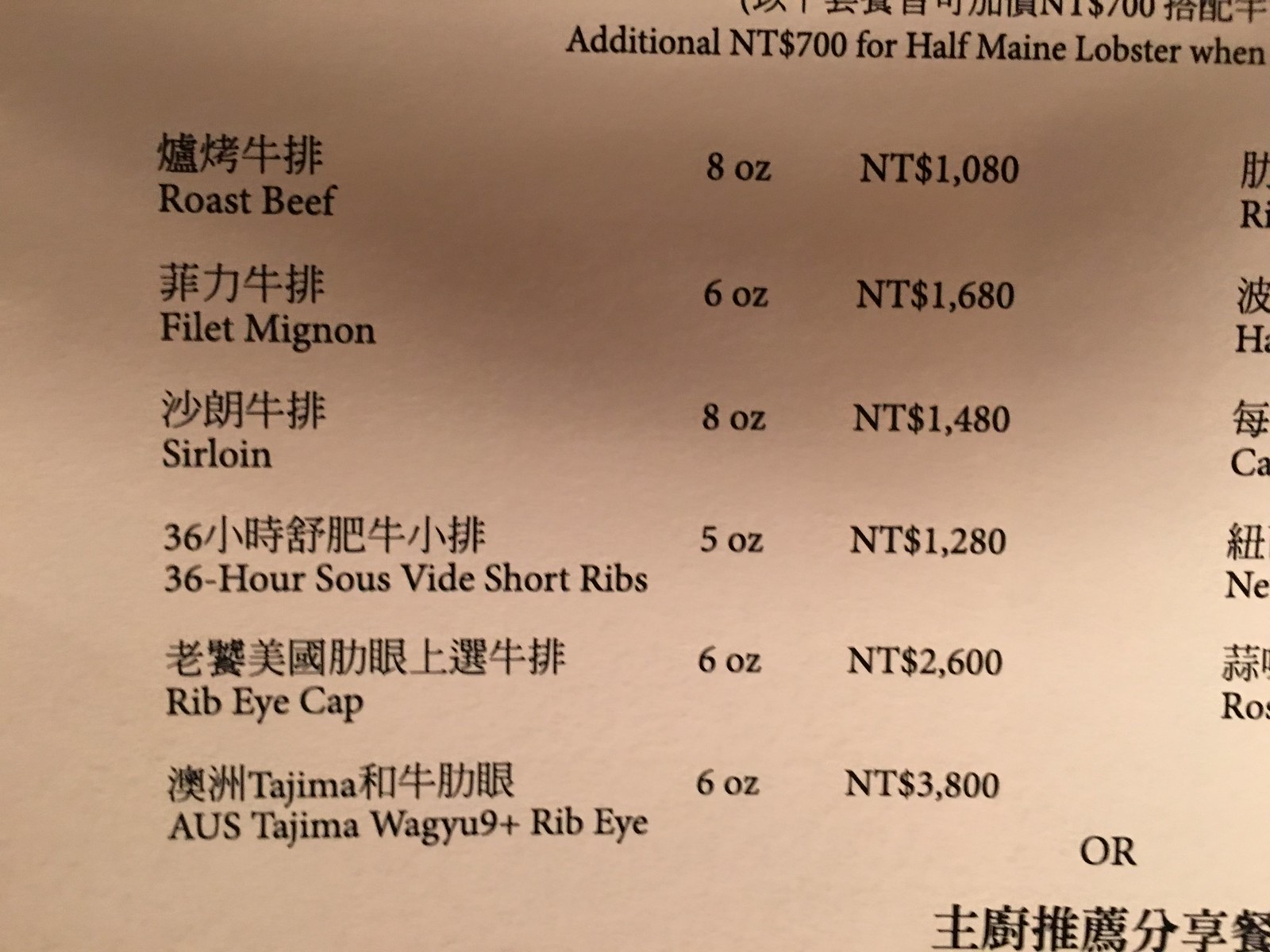This image captures a menu from a Chinese restaurant, meticulously detailing a variety of meat dishes alongside their respective Chinese names, portion sizes, and prices. 

At the very top of the menu, an incomplete entry mentions an additional charge of NT $700 for what appears to be a specialty lobster dish. 

The menu items listed proceed as follows:

- **Roast Beef**: Displayed in both Chinese characters and English, this dish offers an 8-ounce portion priced at NT $1080.
- **Filet Mignon**: Listed in Chinese characters followed by the English translation, the filet mignon is offered in a 6-ounce portion for NT $1680.
- **Sirloin**: This item, also accompanied by its Chinese name, provides an 8-ounce portion at NT $1480.
- **Sous Vide Short Ribs**: Indicated in Chinese characters, the 5-ounce portion of arrow sous vide short ribs is available for NT $1280 and is labeled with the number “36”.
- **Ribeye Cap**: Detailed first in Chinese and then in English, the 6-ounce ribeye cap is priced at NT $2600.
- **Tejima Wagyu**: Listed in Chinese followed by "AUS Tejima Wagyu 9+ Ribeye," this premium meat option offers a 6-ounce portion for NT $3800.

The menu's right side is partially cut off, suggesting additional entries and details are not fully visible, leaving some specifics incomplete.